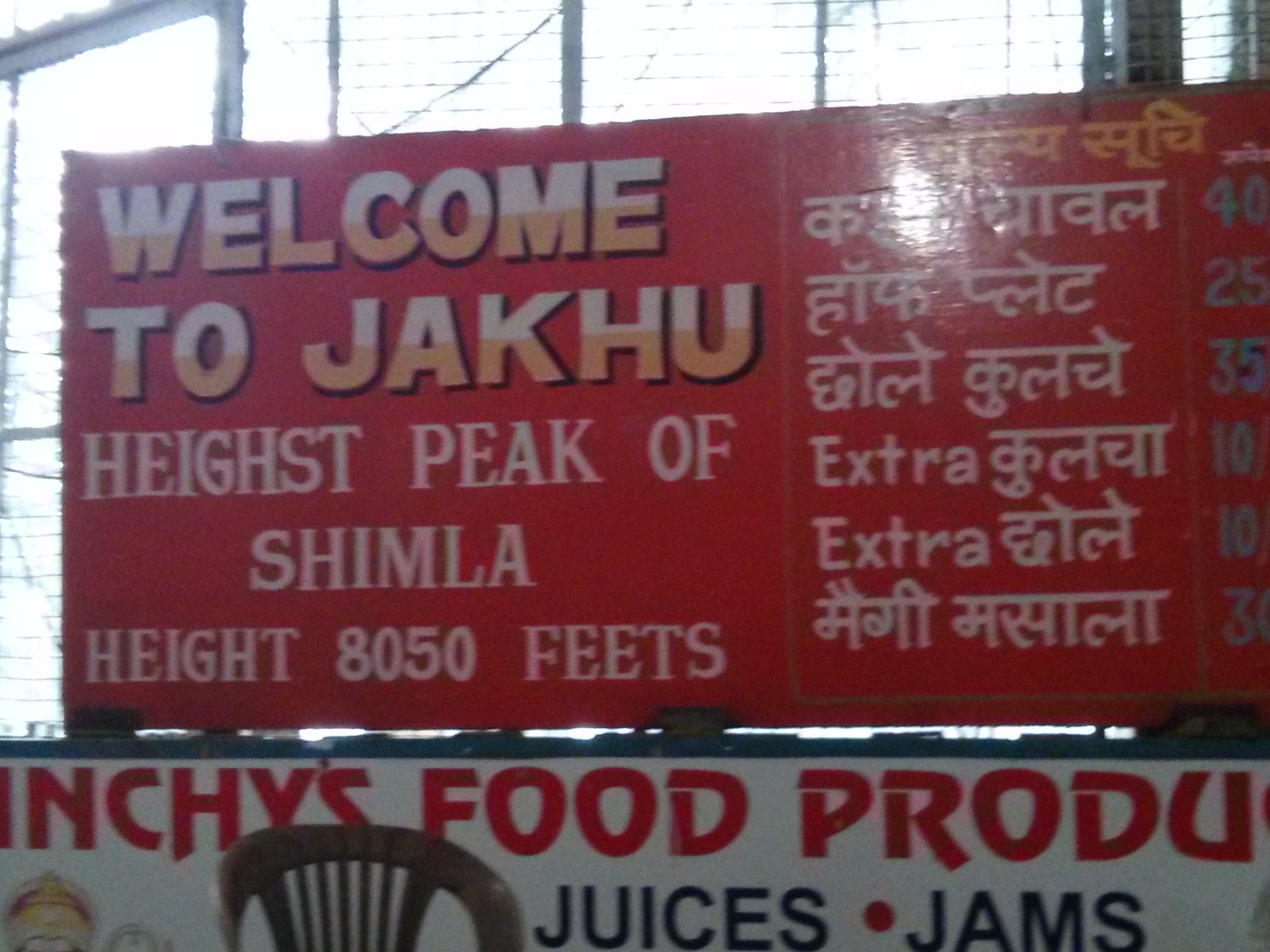The photograph features a vividly red outdoor sign illuminated by beaming sunlight. Positioned at the left side of the sign, the text reads "Welcome to Jakhu," spelled out in white and orange letters with a black outline. Below, it mentions "Highest peak of Shimla, height 8,050 feet," although "highest" is misspelled as "H-E-I-G-H-S-T." On the right side of the sign, there's text in a different language, alongside the English word "extra." Adjacent to this, blue font lists a series of numbers: 40, 25, 35, 10, 10, and 30. Beneath all of this, a separate white sign with red lettering advertises "Inchie's Food Products, Juices, Jams." The area around the sign appears to be an outdoor location enclosed by a high wire fence, suggesting it is a public or recreational space.